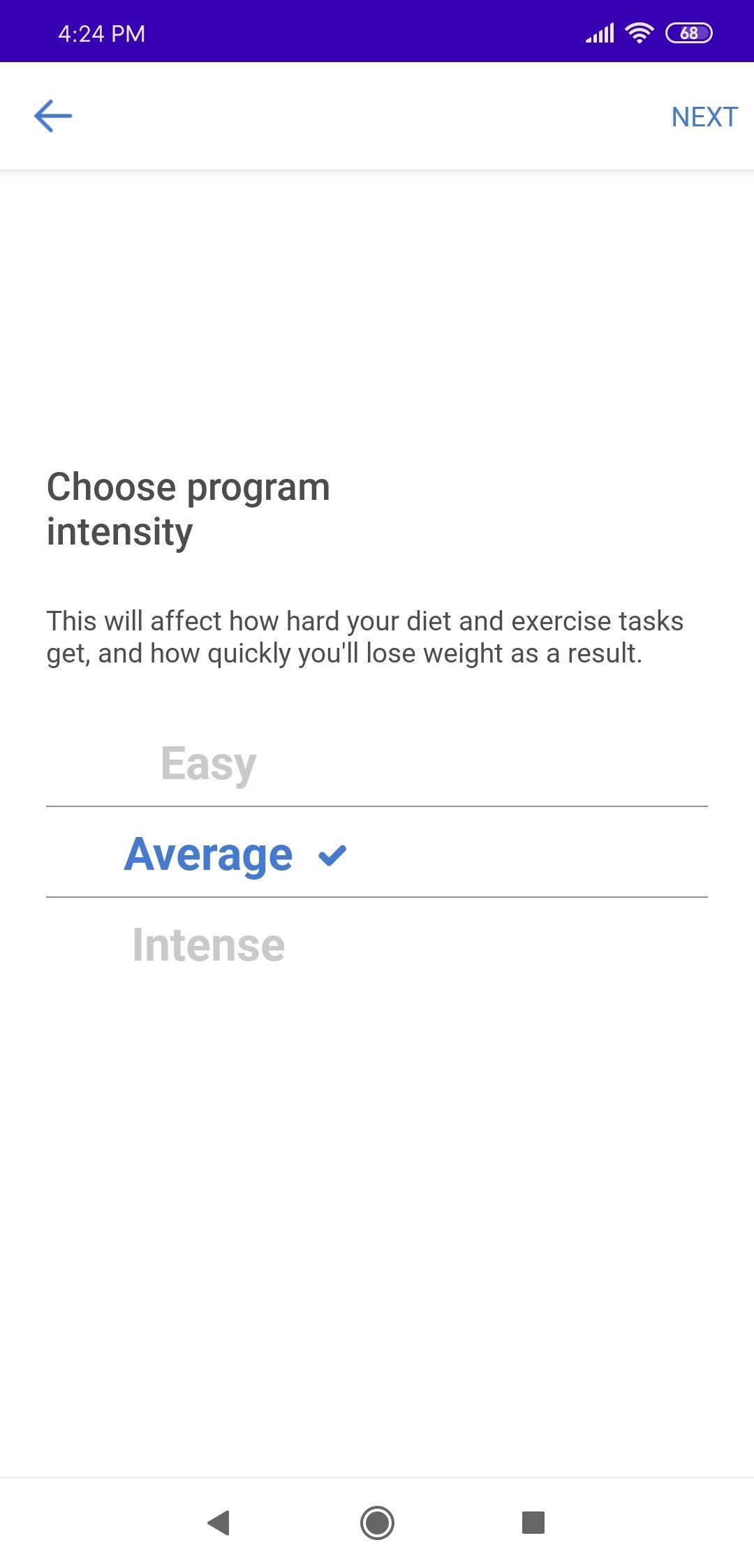This screenshot captures a mobile app's exercise page, featuring a clean and straightforward design. The background is white, while the header area is highlighted with a purple accent color. At the center of the screen, the text "Choose Program Intensity" is prominent, with "Choose Program" on the first line and "Intensity" on the second. Beneath this header, there's a brief explanatory sentence: "This will affect how hard your diet and exercise tasks get and how quickly you'll lose weight as a result."

Below the description is a scrollable menu with three options for program intensity. The top option, "Easy," is displayed in light gray, indicating it is not selected. This is followed by a thin horizontal line. The middle option, "Average," is the selected choice, shown in blue with a corresponding blue checkmark to its right. Another thin horizontal line separates this from the third option, "Intense," which is again in light gray to denote it's unselected.

At the bottom of the screen, a thin dividing line sits above three central navigation buttons: a play button with a left-facing point, a record button illustrated as a circle inside an outer circular outline, and a stop button represented by a square.

In the purple accent area at the top, the time is displayed as 4:24 p.m. in white text. The UI also shows full cell strength with five bars, full Wi-Fi strength, and a battery charge level of 68%, depicted as an oval rather than the traditional battery symbol. Below this, a minimal navigation bar includes a blue back arrow on the left and the text "NEXT" in all caps and blue on the right, separated by a light gray dividing line.